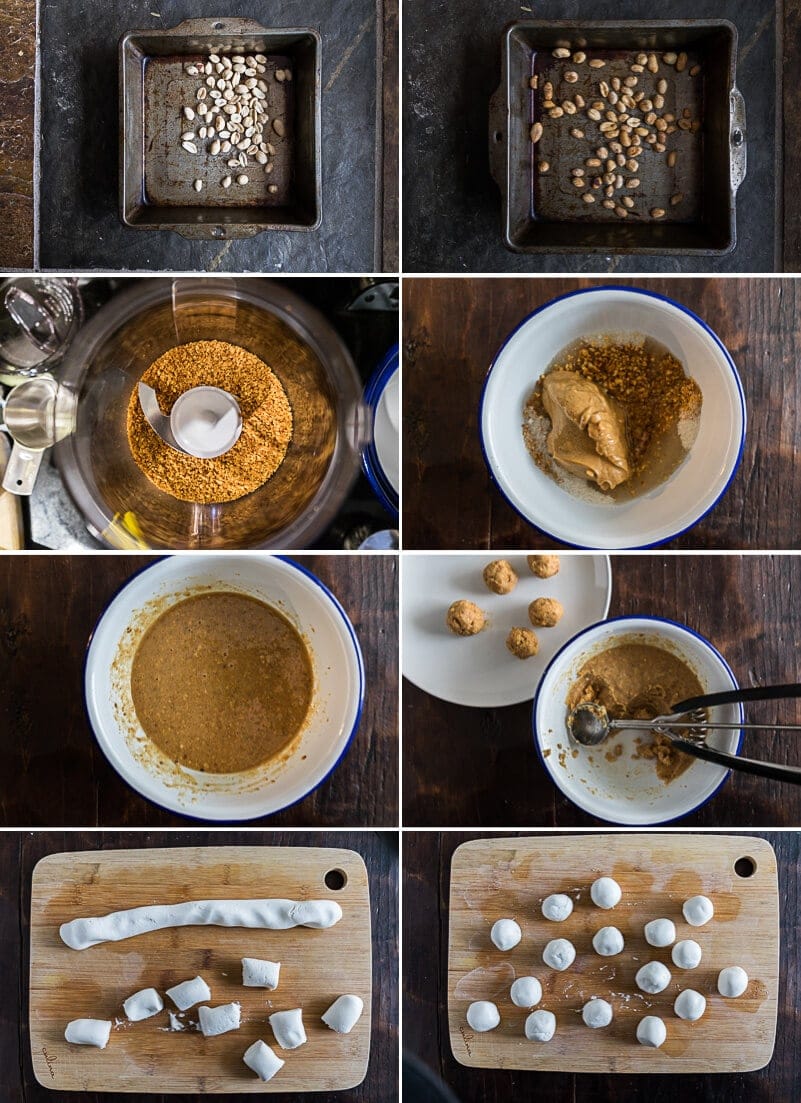This is a series of process photos for a rice ball recipe. 

The topmost images depict dried seeds, potentially nuts, inside a metal pan. The first image shows the nuts in a raw white form, while the second image shows them browned, perhaps after being roasted in an oven. 

In the second row, the left image shows these browned nuts being ground in a food processor. The right image showcases the ground nuts combined with what seems to be a mixture involving a piece of chicken or chicken stock and flour.

The third row depicts a close-up of a liquid mixture, possibly the combined ingredients after blending. Next to it, there is an image displaying the process of using a melon baller to shape the flour mixture into small rice balls.

The bottom row consists of two pictures. The left image shows a long string of dough being sliced on a cutting board. The final image on the right illustrates the dough pieces shaped into round, white balls, placed on a cutting board.

These step-by-step images effectively guide viewers through the process of making rice balls, from preparing the nuts to shaping the dough into balls.